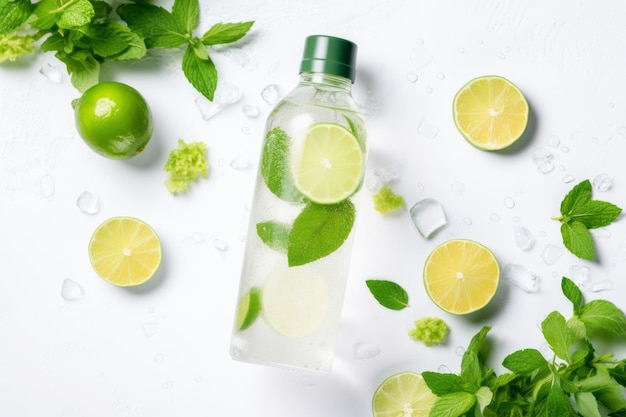This is a detailed photograph of a lime and mint infused water bottle set against a pristine white background. The focal point of the image is a clear plastic bottle with a green cap, situated centrally. Inside the bottle, there are two lime halves and several mint leaves, giving the water a slight greenish tint. The composition is artistically arranged with numerous ice pieces scattered across the white surface.

In the upper left corner, a whole glossy lime sits beside a half-cut lime and a cluster of mint leaves. The bottom right corner mirrors this arrangement with more mint leaves and three additional lime slices. Scattered water droplets and the melting ice contribute to the refreshing theme of the photograph. The image captures the vibrant green hues of the limes and mint contrasted against the stark white background, emphasizing the fresh and invigorating essence of the infused water.